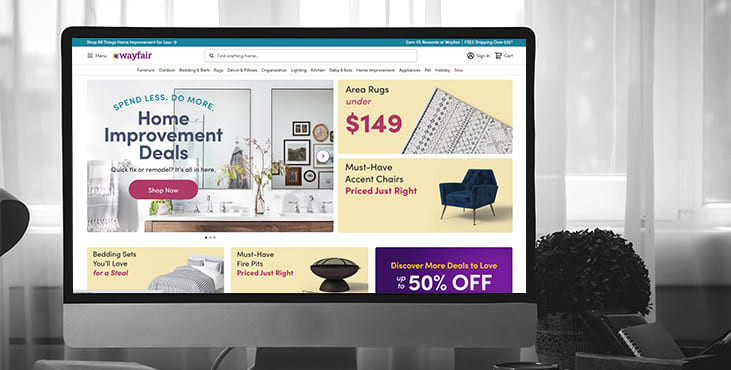A black and white photograph captures a minimalist desk setup positioned in front of a window draped with sheer curtains. On the dark-hued desk, a wide variety of items can be seen, including a small spiral-bound notebook, a fuzzy-looking potted plant, a pair of glasses, and a tray that appears to hold the notebook and possibly a cell phone. However, the central focus of the image is a widescreen monitor with a silver bar at the bottom and a black bezel around the screen.

The monitor prominently displays the homepage of the Wayfair website, which is divided into various tiles showcasing different products. The largest tile features an image of a bathroom with two sinks and mirrors, accompanied by text that reads, "Spend Less, Do More. Home Improvement Deals. Quick fix or remodel, it's all in here." Below this text is a purple button labeled "Shop Now." To the right of this main tile are two smaller tiles: one advertising "Area rugs under $149" with a geometric-patterned rug displayed, and another promoting "Must have accent chairs, priced just right," featuring an image of a sleek black chair with long legs.

At the bottom of the screen, partially clipped by the monitor's edge, is a bar containing three more promotion boxes. The first box highlights "Bedding sets you'll love for a steal," with an image of a striped bedspread. The middle box features "Must have fire pits, priced just right," showing a unique, interconnected double-hemisphere fire pit. The last box is a purple banner that reads, "Discover more deals to love, up to 50% off."

The photograph exudes a clean and organized workspace vibe, emphasizing the online shopping experience on Wayfair's sleek, user-friendly interface.